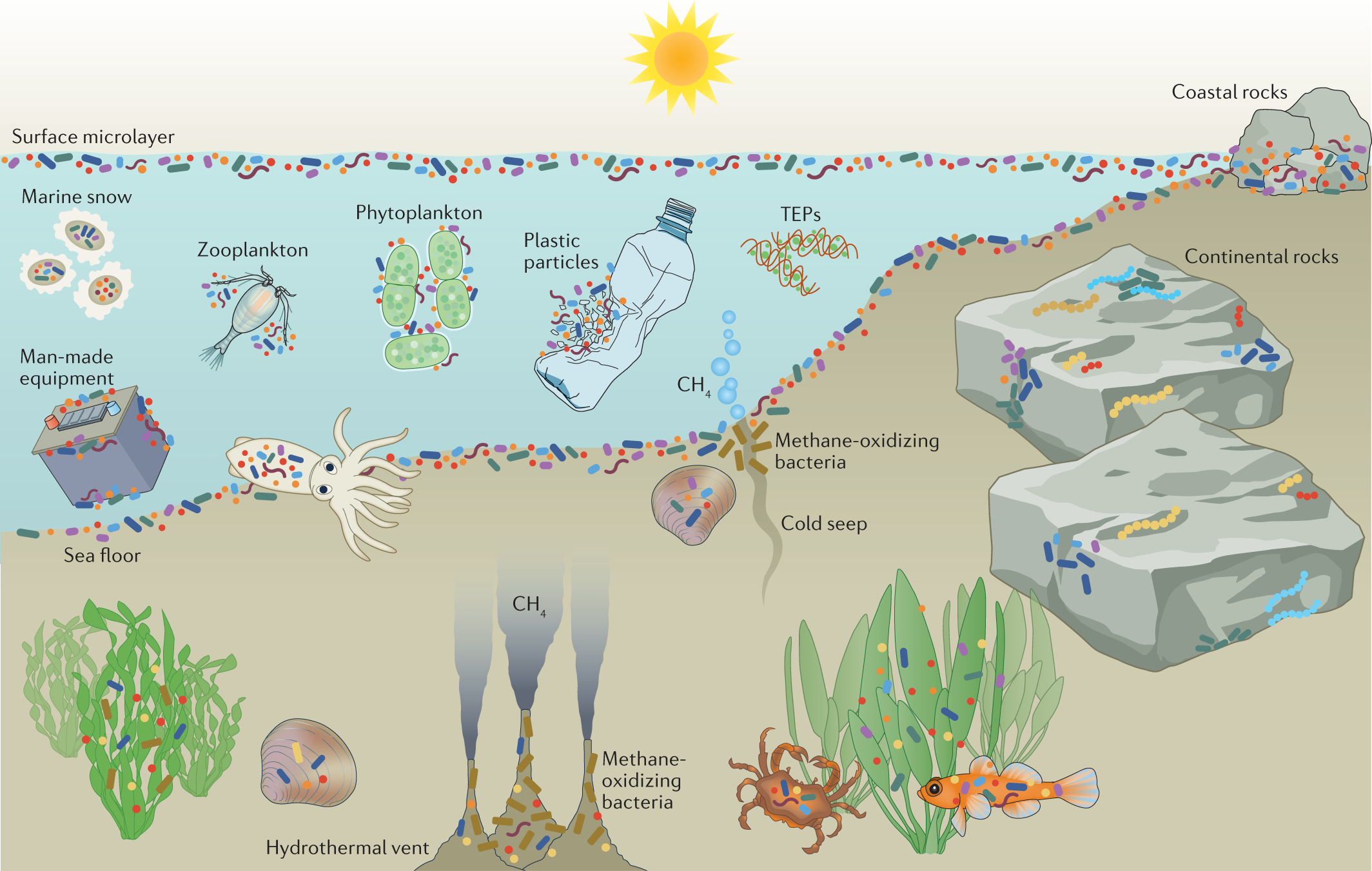The image is an educational diagram illustrating both the water body and the surrounding ground area, focused on the ocean and its various layers. At the top center of the image, a yellow sun is depicted, shining down on the ocean surface, which features a “surface microlayer” rich with plastic particles. The water body, colored blue, dominates the upper portion of the image and is bordered by coastal and continental rocks labeled accordingly. 

Within the water, various components are meticulously labeled with black text, illustrating both natural and man-made elements. Marine snow, small organic particles, drifts down through the water, while zooplankton and phytoplankton, both shown with plastic particles adhering to them, highlight the impact of pollution. The diagram also includes man-made debris such as plastic bottles and other discarded items, showcasing their hazardous effects on marine life.

Further down in the diagram, the seafloor is detailed with elements such as a hydrothermal vent, which emits CH4 (methane) and features methane-oxidizing bacteria. Other depicted elements include green algae, a squid, a crab, and orange fish. Cold seeps and underwater volcanic activities are also indicated, illustrating their role in oceanic ecosystems. Overall, the diagram captures the complex interplay of natural and man-made factors within oceanic and coastal environments.